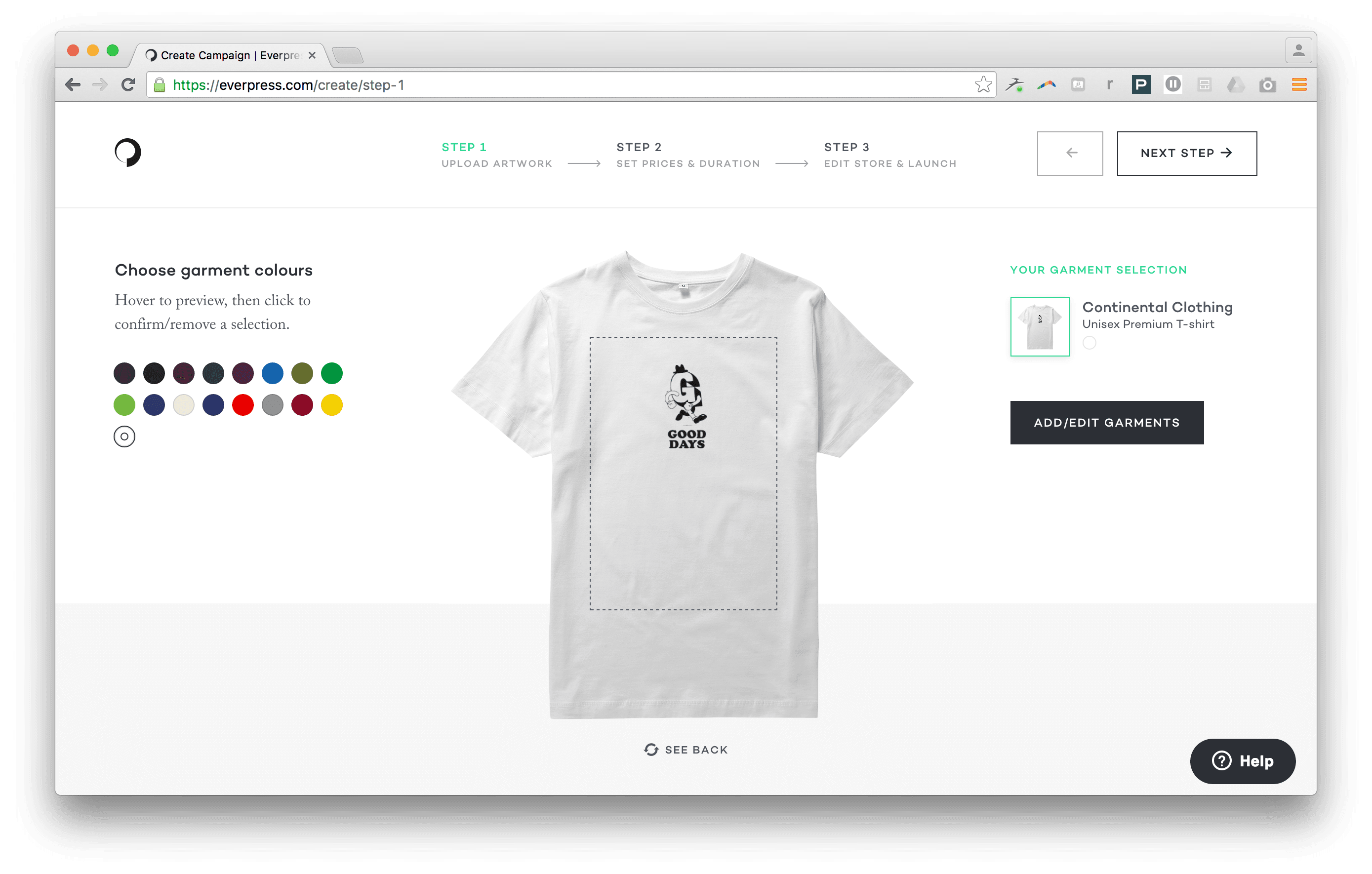**Detailed Screenshot Description:**

The image depicts a screenshot from a website page in landscape mode with a light gray background. 

**Upper Section:**
- The upper left corner features three colored dots: red, orange, and green.
- Adjacent to the dots is a tab labeled "Create Campaign - EverPress."
- The second row includes a back arrow, a refresh button, and a URL field. In the URL field:
  - A green shopping bag icon is visible.
  - The URL entry shows "https://everpress.com", indicating a secure connection.
- To the right of the URL, there are various icons, including a "P" inside a square and three orange horizontal stripes towards the far right.

**Steps Section:**
- The row right below the URL field contains:
  - A black icon on the left side.
  - Text in green illustrating the steps to create a campaign on EverPress:
    - Step 1: Upload Artwork
    - Step 2: Set Prices and Duration
    - Step 3: Edit Store and Launch
- Below these steps, two buttons are present:
  - On the left, a back button.
  - On the right, a boxed button labeled "Next" in black.

**First Column (Left Side):**
- "Choose Garment Colors" is suggested, encouraging users to hover to preview and click to confirm or remove selections.
- A variety of color options are displayed including:
  - Multiple blacks,
  - Blue, olive green,
  - Light green, blue, white, another shade of blue, red, gray, maroon, and yellow.

**Second Column (Center):**
- The highlighted t-shirt design currently reads "Good Days." 

**Third Column (Right Side):**
- This column, labeled in green, is titled "Your Garment Selection."
- A green-highlighted box showcases the t-shirt, labeled "Continual Clothing Unisex Premium T-shirt."
- Below this box is a black button labeled "Edit Garments" for further customization.
- In the bottom right-hand corner of the page is a black help button.

**Overall Layout:**
- The layout is structured and categorized clearly into sections providing users with step-by-step navigation to create and customize their garments on the EverPress platform.